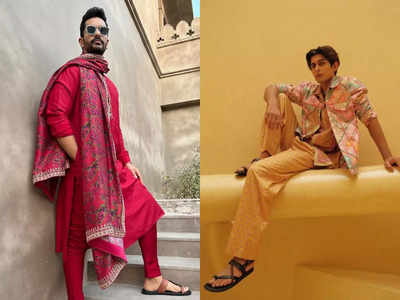The image features two side-by-side photos showcasing eclectic male fashion. On the left, a Caucasian man with fluffy black hair and a short beard stands outdoors against a cement stairway next to a gray wall, possibly part of a temple. A bush, a glimpse of the sky, and a fence are visible in the background. He sports a bold ensemble consisting of a long red dress paired with red leggings, a floral ethnic-looking scarf draped over one shoulder, and sandals. He completes his look with sunglasses, giving an air of sophisticated eccentricity. 

The right photo also depicts a Caucasian man with short brown hair. He is sitting against an entirely yellow backdrop, on what appears to be a yellow bench. His attire includes a vibrant floral print jacket in shades of pink, blue, and white, contrasting sharply with his bright yellow pants. Black sandals adorn his feet. The overall composition of both images emphasizes a striking blend of colors and cultural attire, spotlighting innovative and unconventional fashion choices for men.